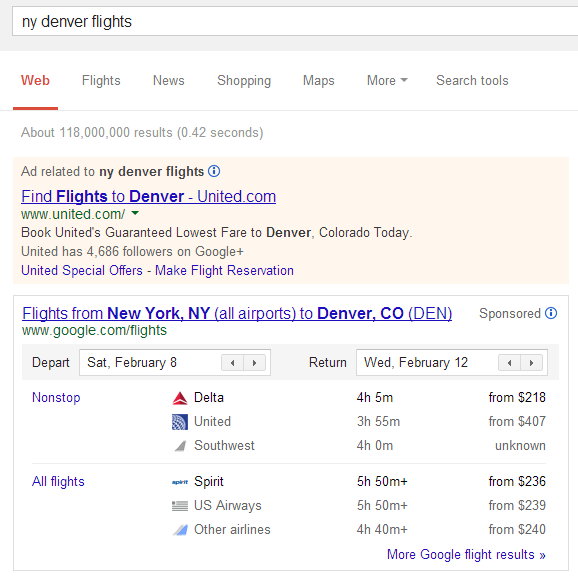The image captures a screenshot of a web page where someone searched for "N.Y. Denver Flights." At the top, the web search category is highlighted in red. The navigation bar below includes various options such as Flights, News, Shopping, Maps, More, and Search Tools. The search results page shows the total number of results and the time taken to generate them in parentheses.

An advertisement prominently displayed at the top promotes flights to Denver from united.com, offering a guaranteed lowest fare if booked today. It also mentions United Airlines' presence on Google+ with 4,685 followers and highlights special offers, along with options to make flight reservations.

Details at the bottom of the page reveal the user’s specified travel dates: departing on Saturday, February 8th, and returning on Wednesday, February 12th. Various flight options are listed, including a nonstop Delta flight lasting four hours and five minutes, starting at $218. Another option shows a United flight with a duration of three hours and fifty-five minutes, costing $407. Additional flight alternatives are available as the viewer scrolls down the page.